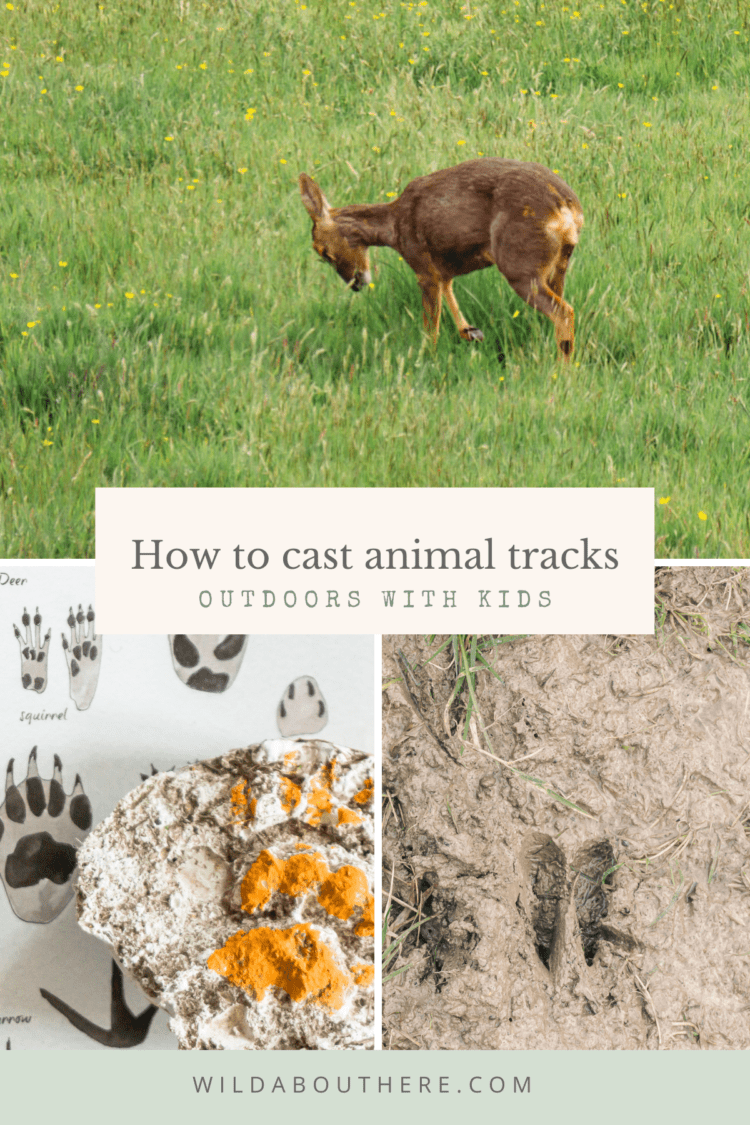This image appears to be a book cover or a page from a website, likely an advertisement for a guide on tracking animals. The focal point is a white rectangular banner in the center, boldly titled "How to Cast Animal Tracks Outdoors with Kids" with supplementary text below it. The layout consists of three photos. The top photo captures a serene field with tall, bright green grass adorned with sporadic yellow wildflowers. Grazing in the middle of this field is a baby deer, also known as a fawn, distinguished by its dark brown fur with lighter patches and head down, suggestively feeding.

The bottom of the cover is divided into two side-by-side images. On the left, a black and white graphic displays various animal paw prints. Superimposed on this graphic is a plaster cast of an animal track, painted in orange to highlight the print. The right-hand image showcases a sepia-toned view of dirt with a pair of dark hoof prints, likely deer tracks, accompanied by scattered green leaves. 

A light gray banner stretches across the bottom of the image, containing the text "wildabouthere.com," indicating the source or creator of the content.